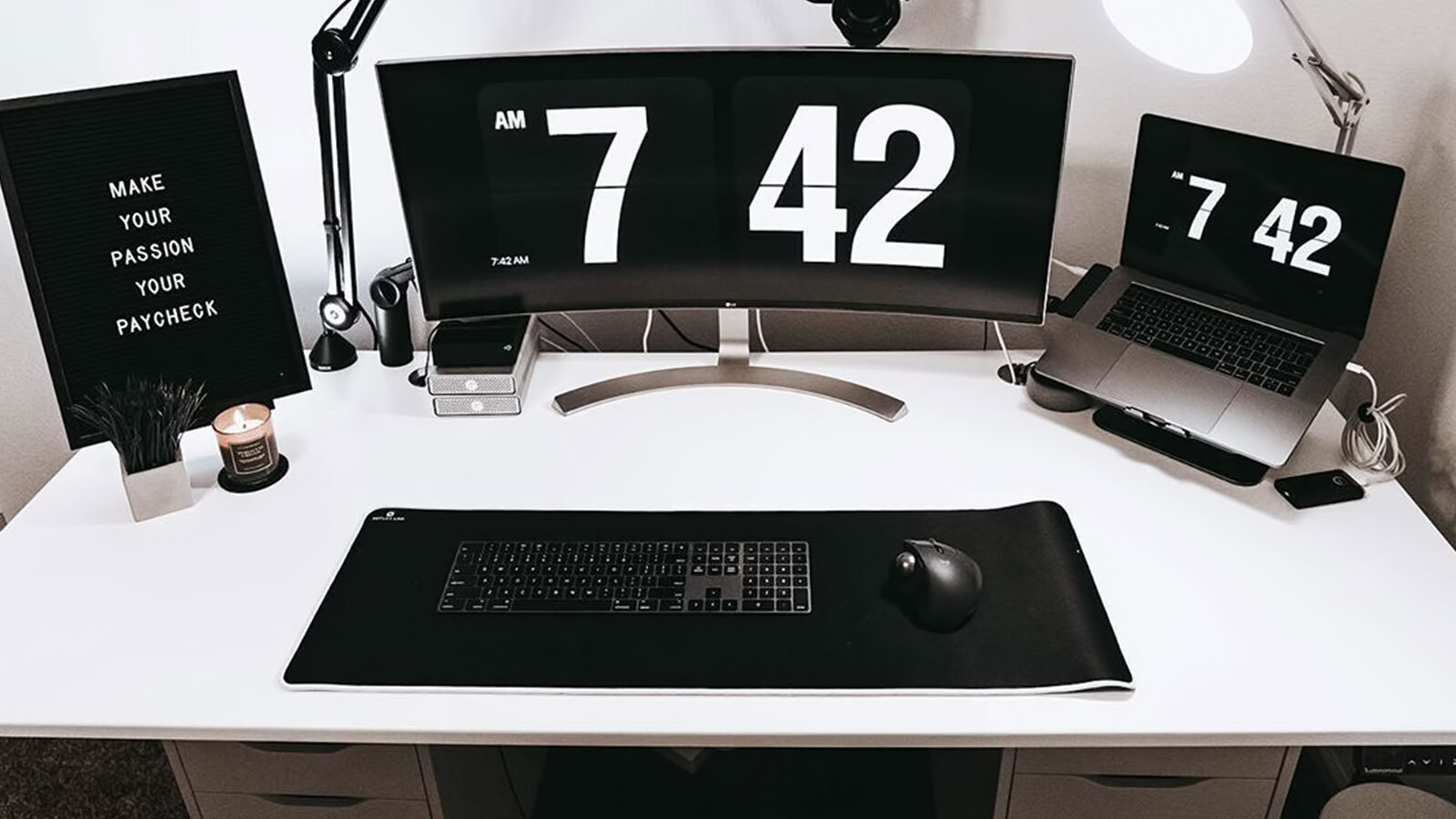The photograph depicts a meticulously organized computer desk setup. The desk features a flat white surface supported by a gray frame, with drawers on both the left and right sides, and a space underneath for legs or a chair. Situated on the desktop is an inspirational quote framed in black, reading "MAKE YOUR PASSION YOUR PAYCHECK" in white capital letters.

The workspace includes a variety of items: a small potted plant, a candle, a mouse and keyboard placed on a desk mat, a computer monitor, and a laptop positioned on an angled platform. A microphone on a gimbal arm is also present. Additionally, a Wi-Fi router or hard drive box can be seen. The computer monitor and laptop both display the time as 7:42 AM. Dominant colors in the image are white, black, and gray, contributing to a clean and modern aesthetic.